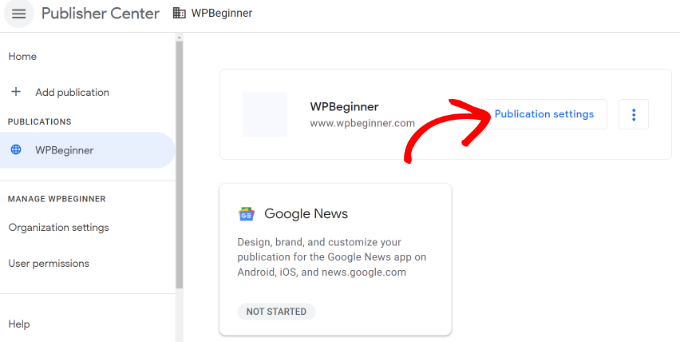The image depicts a snapshot of the Publisher Center interface for "WP Beginner". At the top, there's a gray circular icon containing three horizontal lines stacked vertically. Next to it, the text reads "Publisher Center - WP Beginner" with a horizontal line running beneath it. On the left side of the interface, there's a vertical column featuring a scroll bar on the right. The column's options include "Home" and "Add Publication," followed by a section labeled "Publications."

Within this section, there's a light blue box titled "WP Beginner," accompanied by a horizontal line underneath it. Below this, the options listed are "Manage WP Beginner," "Organization Settings," "User Permissions," and "Help," with corresponding horizontal lines separating each option. 

On the right side of the interface, a larger gray square is displayed with the text "WP Beginner - www.wpbeginner.com" written to its right. Adjacent is a prominent white button labeled "Publication Settings" in blue text, marked by a red arrow pointing towards it and a vertical ellipsis button to its right. Beneath this, there's another informational box that reads, "Google News Design - Brand and Customize Your Publication for the Google News app on Android, iOS, and news.google.com."